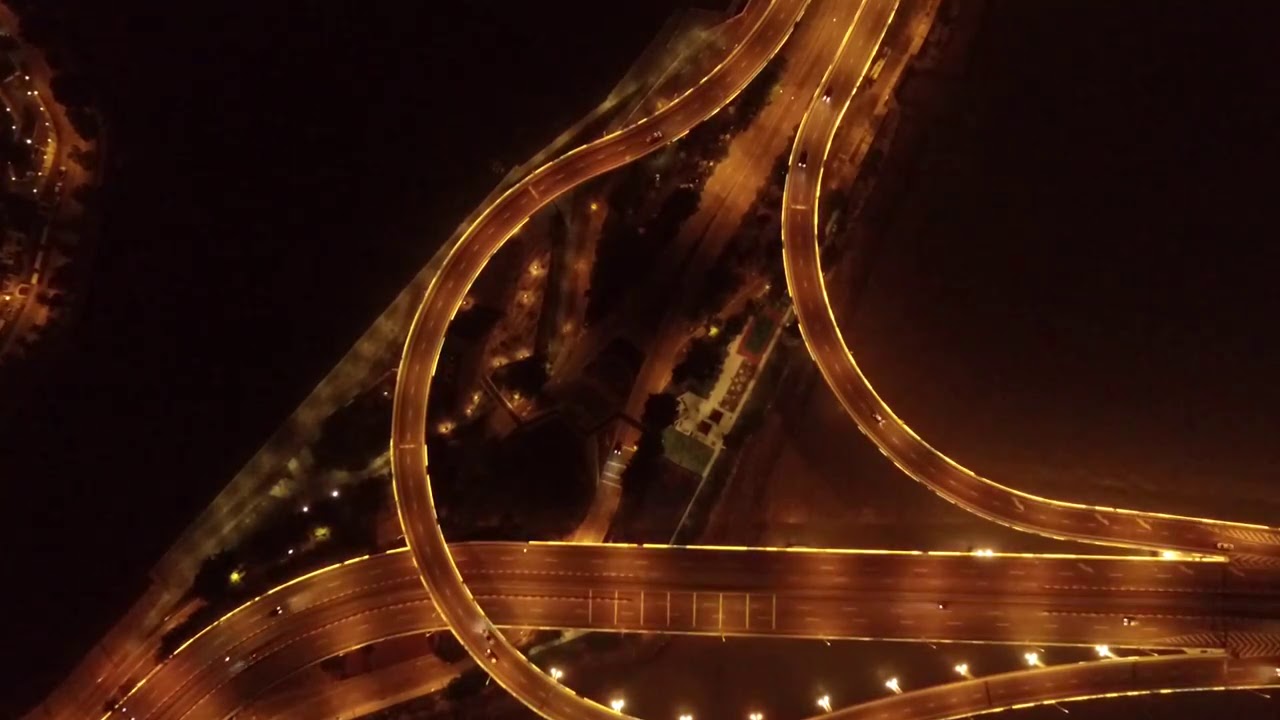The image is a high-resolution, nighttime aerial photograph captured from a significant height, likely using a drone. It showcases a multi-lane freeway with several intersecting and curving pathways. The scene is predominantly dark, illuminated by the consistent glow of streetlights lining the roads and intersection, highlighting the clear and well-defined layout despite the nighttime setting. Vehicles are sparsely distributed across the freeway, with a few tiny cars visible, mainly on the right side of the image. The photograph features trees and scattered illumination sources, contributing to the overall clarity and realism of the scene. The composition, in landscape orientation, is representational, capturing the intricate network of roads and overpasses with great detail and precision.